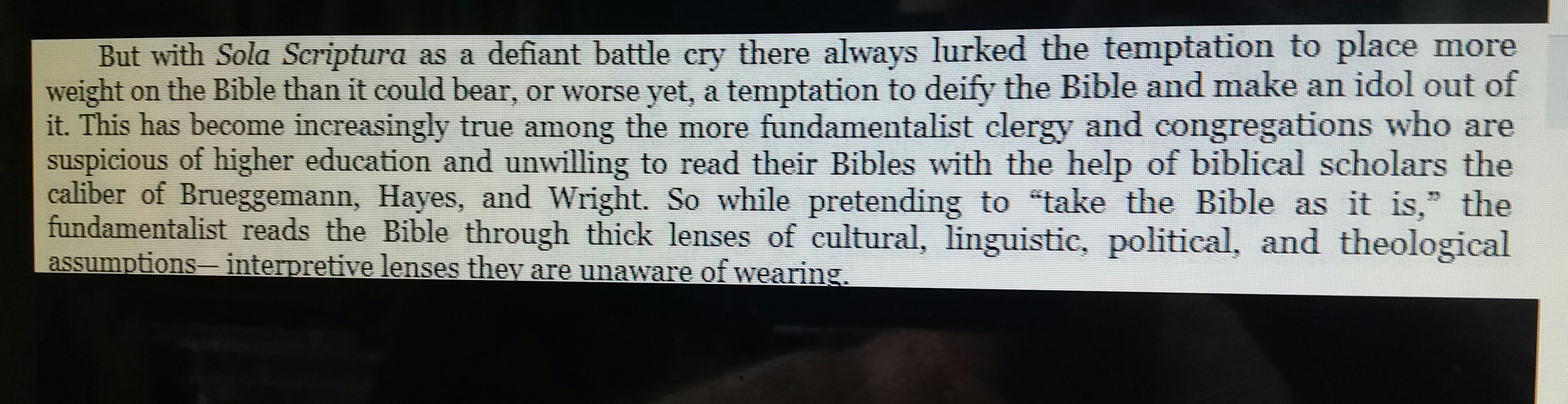The image displays a close-up of a cutout section from a newspaper article, prominently framed by a solid black border. The text is set against a white background, with black lettering that reads: "But with Sola Scriptura as a defiant battle cry, there always lurked the temptation to place more weight on the Bible than it could bear, or worse yet, a temptation to deify the Bible and make an idol out of it. This has become increasingly true among the more fundamentalist clergy and congregations who are suspicious of higher education and unwilling to read their Bibles with the help of biblical scholars the caliber of Brueggemann, Hayes, and Wright. So while pretending to 'take the Bible as it is,' the fundamentalists read the Bible through thick lenses of cultural, linguistic, political, and theological assumptions—interpretive lenses they are unaware of wearing." The overall appearance suggests that this quote was meticulously extracted and mounted on a black background, emphasizing its significance and the critical perspective it conveys on fundamentalist approaches to biblical interpretation.